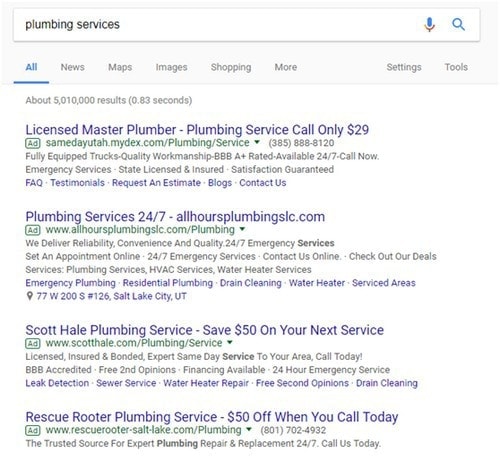A detailed screenshot of a search engine interface on a mobile device displays a user searching for "plumbing services." The interface closely resembles Google's layout. At the top, the search bar includes a search button and a microphone icon. Below the search bar, a gray navigation bar presents several options: 'All' (which is currently selected), 'News', 'Maps', 'Images', 'Shopping', and 'More'. Additionally, 'Settings' and 'Tools' options are located on the right side of the gray bar. The main section of the screen showcases a list of various plumbing service providers, complete with brief descriptions and links to their respective websites.